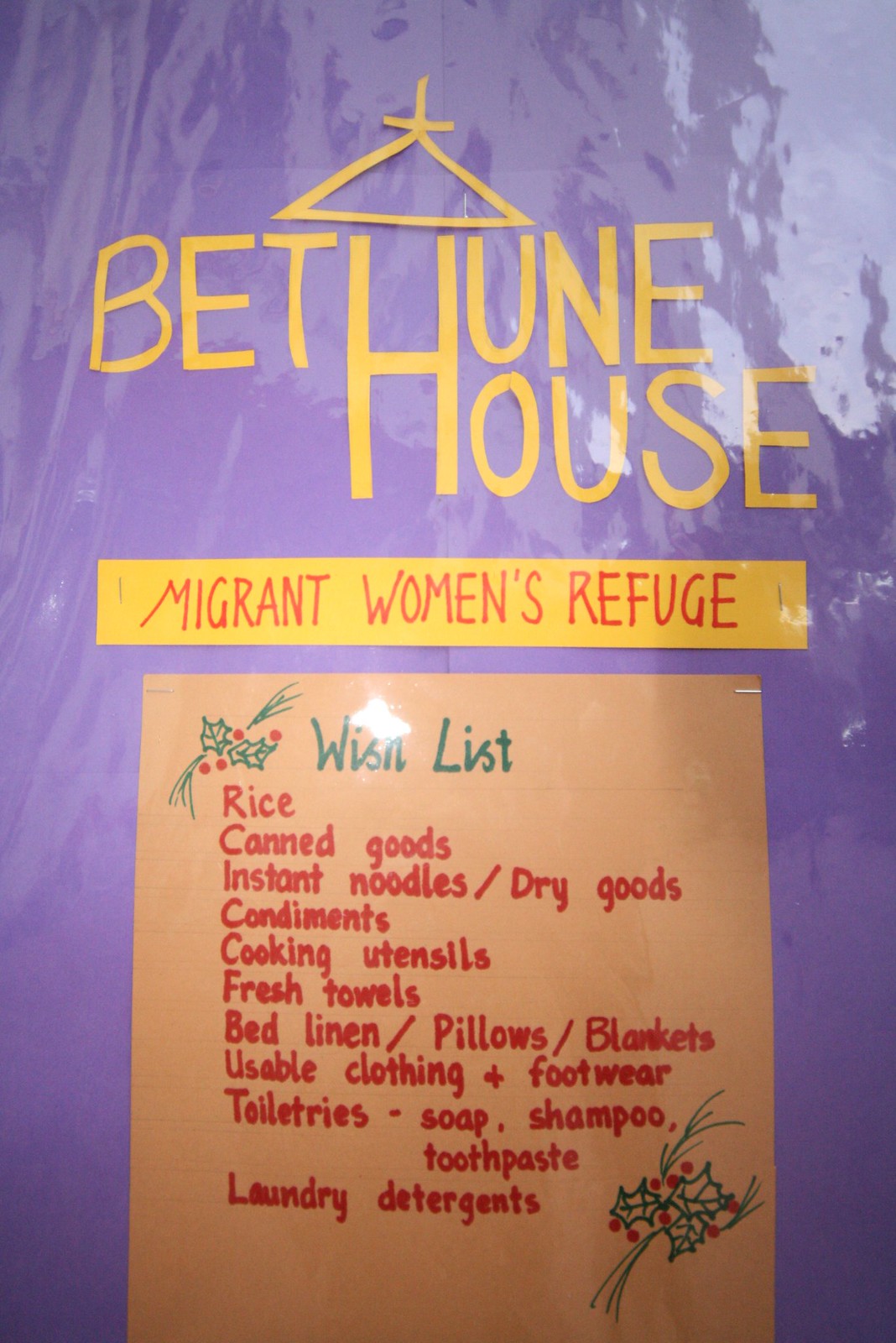The image displays a poster against a blotchy purple background with a prominent glare that suggests it might be behind glass, possibly a window display. At the top, in large yellow letters cut from construction paper, it reads "Bethune House," featuring a joint "H" that merges the words "Bethune" and "House." Above this text, there's a triangle logo with an upside-down cross at its peak.

Beneath the title, there's a red rectangle with bold white letters stating "Migrant Women's Refuge." Directly beneath that, a brown piece of cardboard with green lettering outlines a "Wish List," adorned with holly leaves and berries drawn with markers in the upper left and bottom right corners. The wish list includes the following items in red text: rice, canned goods, instant noodles, dry goods, condiments, cooking utensils, fresh towels, bed linens, pillows, blankets, usable clothing and footwear, toiletries, soap, shampoo, toothpaste, and laundry detergents. The overall aesthetic of the poster gives a handmade and heartfelt appeal, likely aiming to gather donations for a migrant women's shelter.